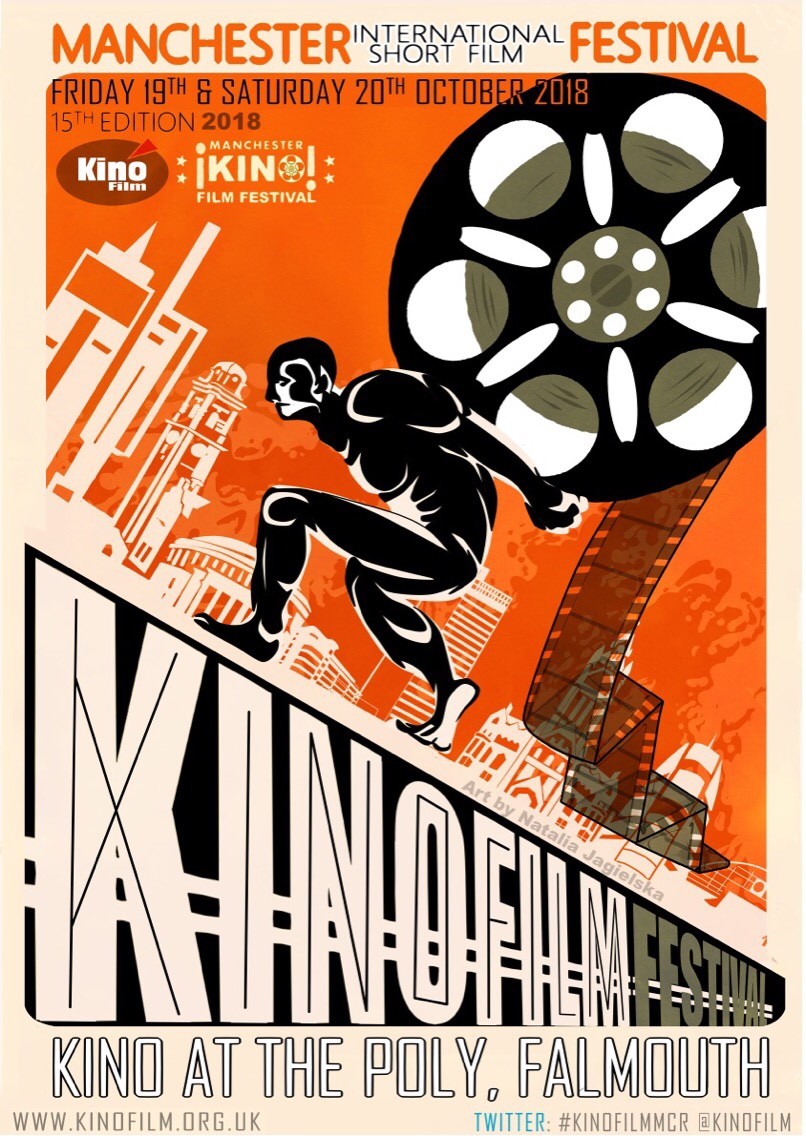The poster for the Manchester International Short Film Festival prominently features an event title at the top in bold black and orange lettering: "Manchester International Short Film Festival." The dates, "Friday 19th and Saturday 20th October 2018," are listed beneath, alongside the indication that it is the "15th edition 2018."

The central visual element is a striking design of a muscular man climbing an incline, carrying a large, unwinding film reel on his back as he struggles uphill. The man is depicted with black skin and white highlights, against a vivid orange background showing a city skyline. The incline he is climbing features the text "Kino Film Festival." Below this, in large block letters, it states "Kino at the Poly Falmouth." Additionally, there is some light gray text that credits the artwork to Natalia Jagielska.

Further text on the poster includes various festival details and social media information, such as "KINDfilm.org UK" and the Twitter hashtag "KINDfilm MCR," making it clear that this is a well-organized and significant event in the UK film scene.